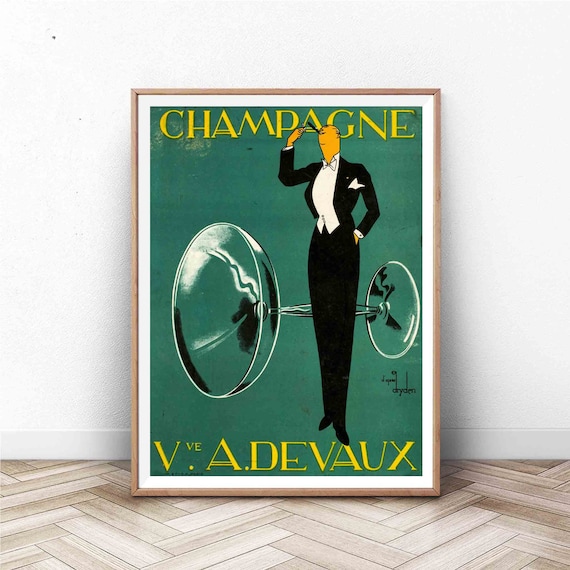The image showcases a framed art print featuring a teal background and vibrant red lettering. The print is titled "Champagne V. A. Duveau" and displays the text "Champagne" at the top in yellow block font, with "V. A. Duveau" at the bottom in a similar style. The artwork portrays a tall, faceless man in a black and white tuxedo, depicted in a cartoonish manner with one hand in his pocket and the other lifting a long cigar to his mouth. He is positioned next to an oversized champagne coupe laying on its side, humorously matching his height. The poster, enclosed in a tan-colored frame with a white border, leans against a white wall upon a light-colored, herringbone-patterned wooden floor.